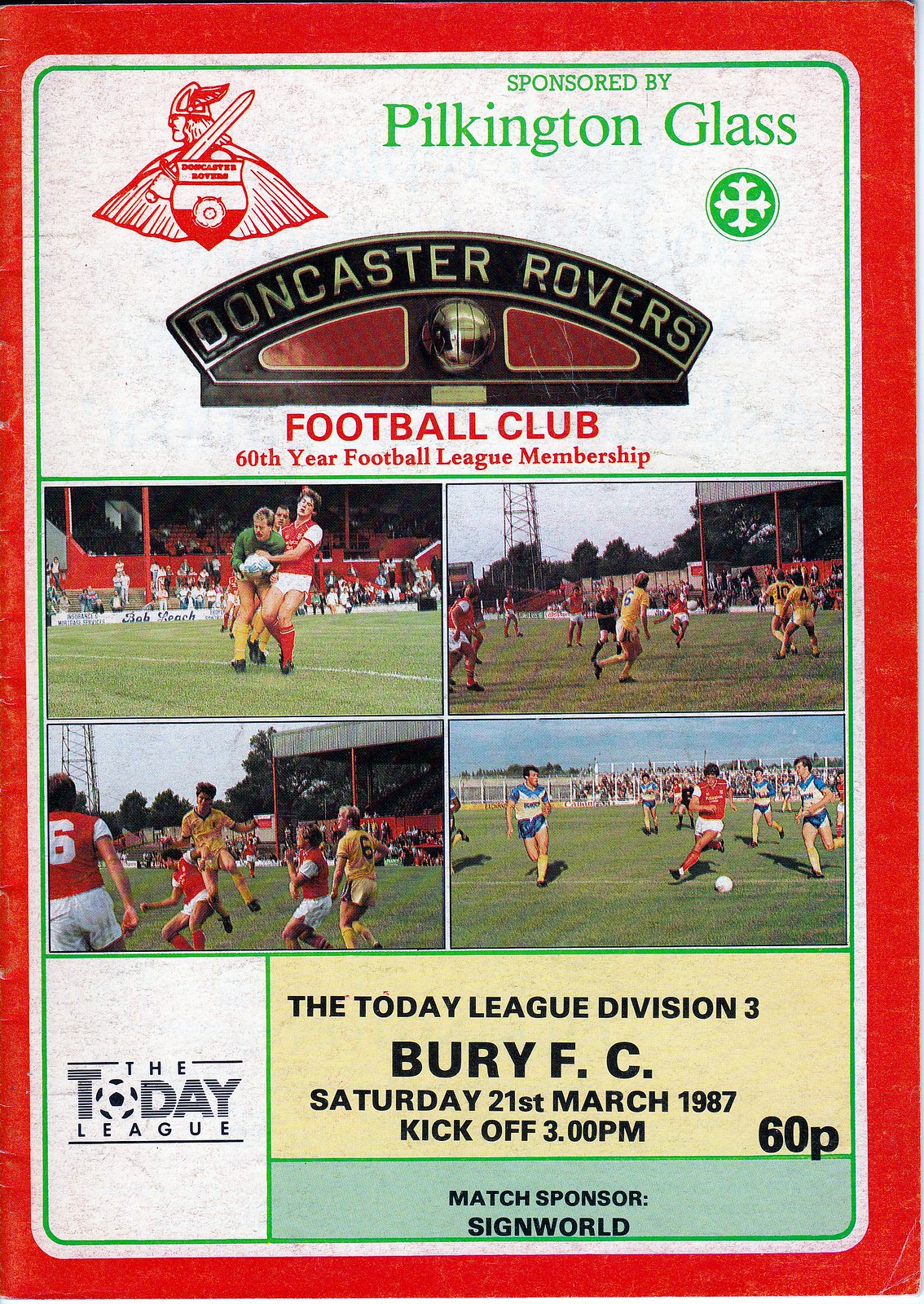This image is the cover of a match program for Doncaster Rovers Football Club, commemorating their 60th year of Football League membership. The cover features a striking red border on all sides, with a thinner red border on the left. The background is predominantly white. In the upper left corner, there is an emblem resembling a Viking with a sword over its shoulder and a green cape. To the right of the emblem, green letters state "Sponsored by Pilkington Glass." Below this, the text reads "Doncaster Rovers Football Club 60th Year Football League Membership" in red. The middle section showcases four action-packed images of live football, arranged in a two-by-two grid. Beneath these images, the text "The Today League Division 3, Bury FC, Saturday, 21st of March 1987, Kickoff 3 p.m." is prominently featured, with "60p" denoting the price. Finally, at the bottom, the match sponsor "Sign World" is acknowledged.